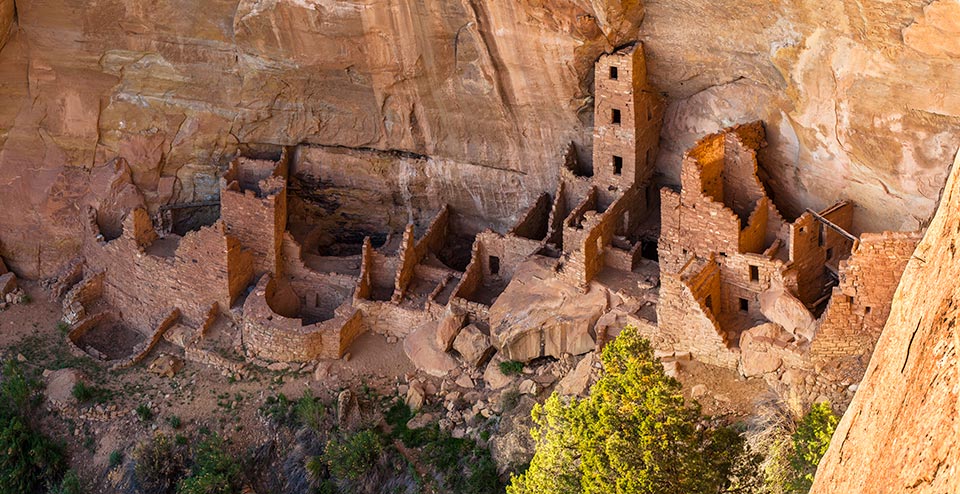This photograph captures an aerial view of ancient ruins built from brown and reddish-brown bricks. The ruins are nestled against and in front of a steep, rocky cliff that dominates the background and right side of the image. The cliff, likely part of a mountain, is a prominent, reddish-brown stone wall. The ruins show various well-defined structures, including large circular areas and raised rectangular or squared towers, many of which are crumbled at the top and missing roofs. One of the towers is notably more intact, standing at least three to four stories high with visible window openings. At the base of the cliff and across the bottom of the image, clusters of green trees provide a natural contrast. The trees on the left side are shrouded in shadow, while those on the right bask in sunlight, appearing bright green. The detailed view from this elevated position reveals signs of human activity, possibly tourists exploring the historic site.